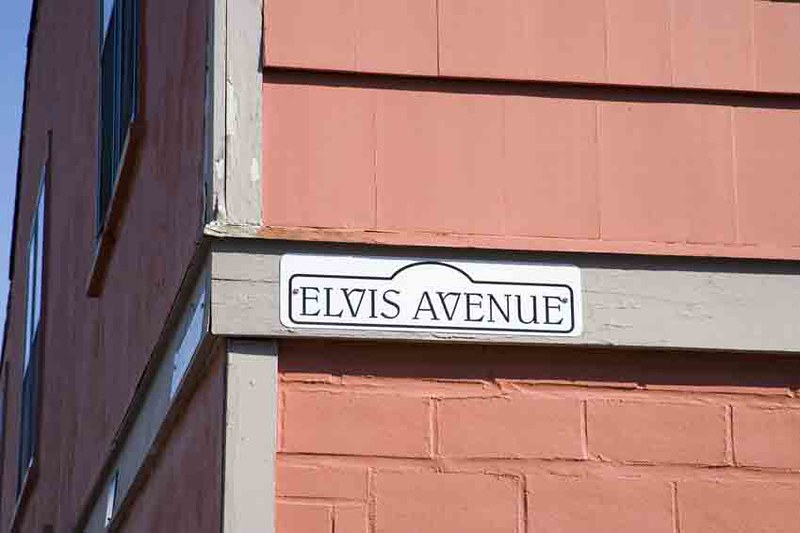The image features a red brick building with a horizontal section painted in peach running across its center. A prominent, gray wooden beam spans this area, bearing a white street sign that reads "Elvis Avenue" in black text. The sign is rectangular with rounded edges and secured with rivets at both ends. On the corner of the building, a similar gray beam extends vertically from top to bottom. Above the horizontal beam on the left side, multiple windows with projecting windowsills are visible. The upper part of the wall showcases cedar shakes painted in the same peach color as the brick, while a sliver of the sky can be seen in the top left corner of the image. The overall setting suggests an urban environment with ambient street sounds.